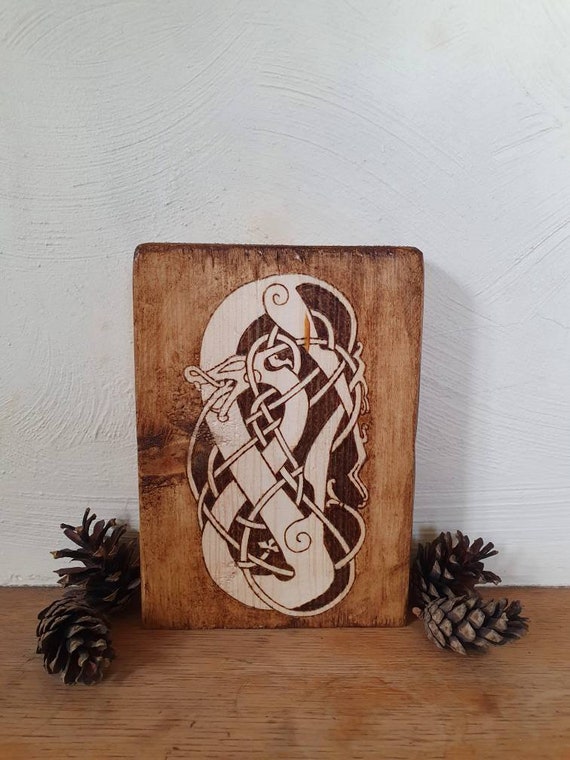The image features a detailed wooden plaque that centers a bold, intricate Norse sea serpent design, either stained or painted with a combination of light tan and dark brown hues. The natural grain, knots, and lines of the wood are visible through the artwork, enhancing the rustic charm. This plaque is set on a wooden table or mantel adorned with four pinecones, two on each side; the left pinecone is upright while the rest are lying on their sides, adding a festive, holiday touch. The backdrop is an off-white, textured plaster wall, with noticeable brush or swish marks, complementing the earthy, handcrafted aesthetic of the scene.